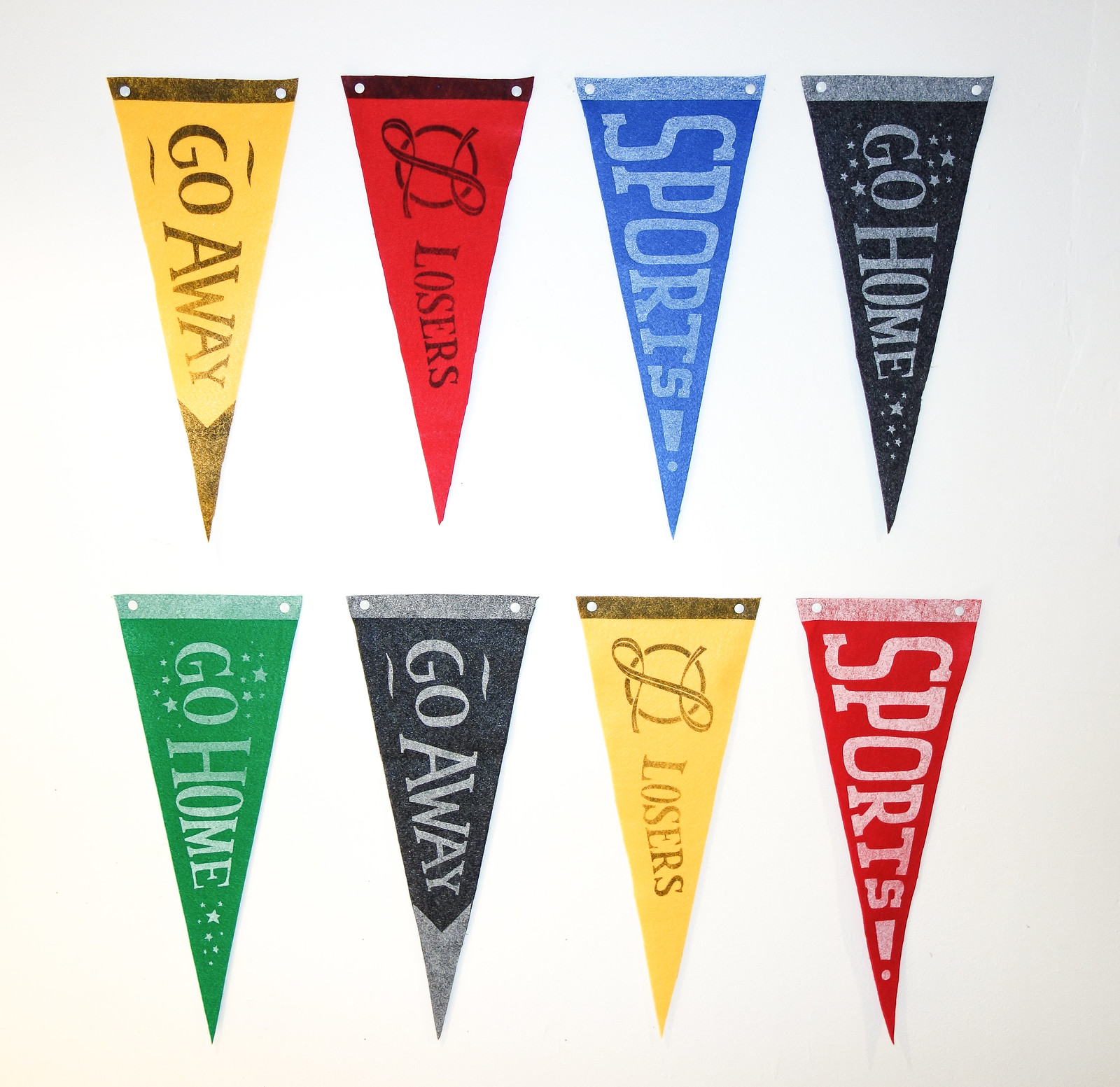The image showcases eight triangular flags arranged on a white background in two rows of four. Each flag, pointing downward, displays various words or phrases. The top row from left to right features: a golden yellow flag with gold text that says "Go Away," a red flag with black text that says "Losers," a blue flag with light blue text that says "Sports," and a denim blue flag with light grey text and tiny stars that says "Go Home." The bottom row from left to right includes: a green flag with white text and small stars that says "Go Home," another denim blue flag with light grey text that says "Go Away," a yellow flag with gold text that says "Losers," and a red flag with pinkish-white text that says "Sports." The flags display repeating themes and colors, often used for decorative purposes.